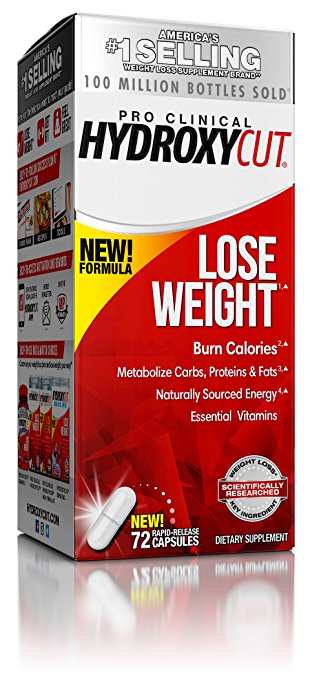This promotional image of a Hydroxycut product showcases a retail box against a reflective white background. The tall, square box prominently advertises Hydroxycut as "America's #1 selling weight loss supplement brand" with "100 million bottles sold." The packaging highlights the product name, "Pro Clinical Hydroxycut," with "hydroxy" in black and "cut" in red. A yellow triangular section at the top proclaims a "new formula," while the red lower portion lists benefits such as "lose weight, burn calories," "metabolize carbs, proteins, and fats," "naturally sourced energy," and "essential vitamins" — all benefits marked with asterisks. An image of a white capsule on the left side is labeled "new" in yellow, indicating the box contains "72 rapid-release capsules." Slightly visible on the side are images of various Hydroxycut products. The detailed design and marketing promises suggest this dietary supplement is intended for retail pharmacy sections, offering a scientifically researched weight loss aid to be used alongside an exercise regimen.